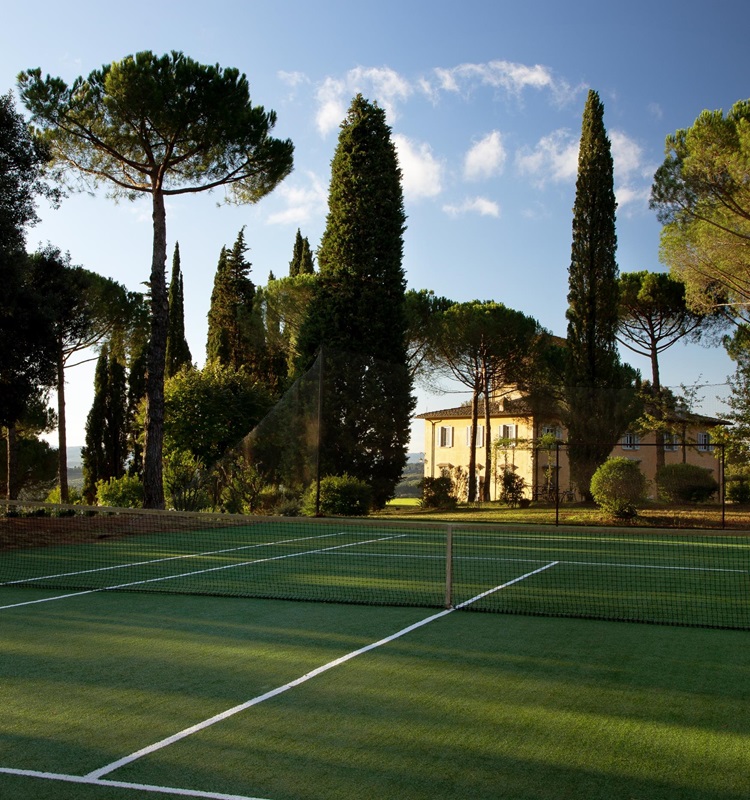This image showcases a meticulously maintained grass tennis court situated on the grounds of a Spanish-style, two-story house with yellow walls. The court, occupying the bottom half of the image, features freshly painted white lines and a waist-high net with a black mesh, supported by wooden stakes. Bordering the court is a chain-link fence, while manicured trees of varying shapes and colors populate the left side, extending towards the background where the house is partially visible. Above the scene, a partly cloudy blue sky adds a serene touch. The photograph, taken from one end of the court looking toward the other, captures a sunny day with late afternoon shadows casting a dramatic contrast on the lush green surface.